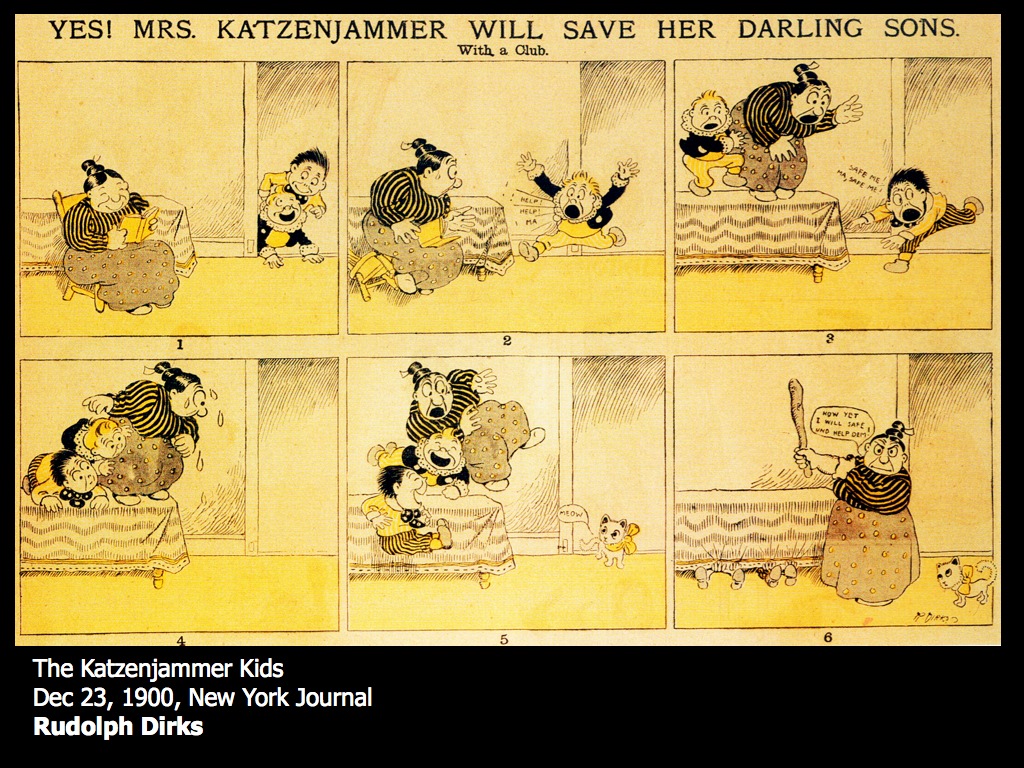This detailed black-and-white comic strip from December 23, 1900, titled "Yes, Mrs. Katzenjammer Will Save Her Darling Sons with a Club," was featured in the New York Journal by Rudolph Dirks. It comprises six square scenes arranged in two rows. At the top, a large black text reads the title, with a smaller subtitle underneath that says "with a club." 

The first panel depicts a woman with dark hair styled in a bun seated calmly, reading a book. Two young boys peek around a corner in the background. In the next panel, one boy dashes into the room, startling the woman and screaming "Help!" 

The following panels show the woman and the first boy standing on a table, visibly frightened. In the subsequent scene, the second boy runs across the room, also screaming for help. The fourth panel reveals all three— the woman and the two boys— huddled on the table, with the woman looking terrified and sweating. 

In the fifth panel, the source of their fright is disclosed as a small kitten with a yellow ribbon walks in, meowing. The boys, previously frightened, now laugh. The final panel shows the woman resolutely pushing up her sleeves, standing back on the ground with a wooden club in her hand, ready to "save" her sons. 

The comic strip concludes with white text on a black border that reads: "The Katzenjammer Kids, December 23rd, 1900, New York Journal, Rudolph Dirks."